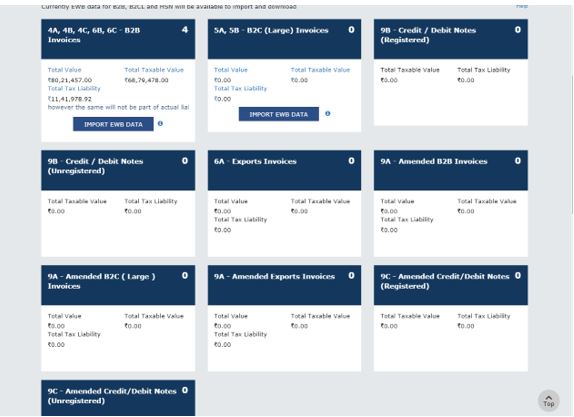This is a screenshot of a website interface designed for managing financial data. The layout consists of multiple cards, each with a blue header and a white body. There are a total of 10 cards arranged in a grid, with three cards per row followed by additional rows scrolling down. Each card displays information related to various types of invoices and credit/debit notices. Specific details shown on the cards include total value, total taxable value, and in some instances, the total tax liability. The background of the website is plain grey, providing a neutral backdrop that makes the blue and white cards stand out prominently.